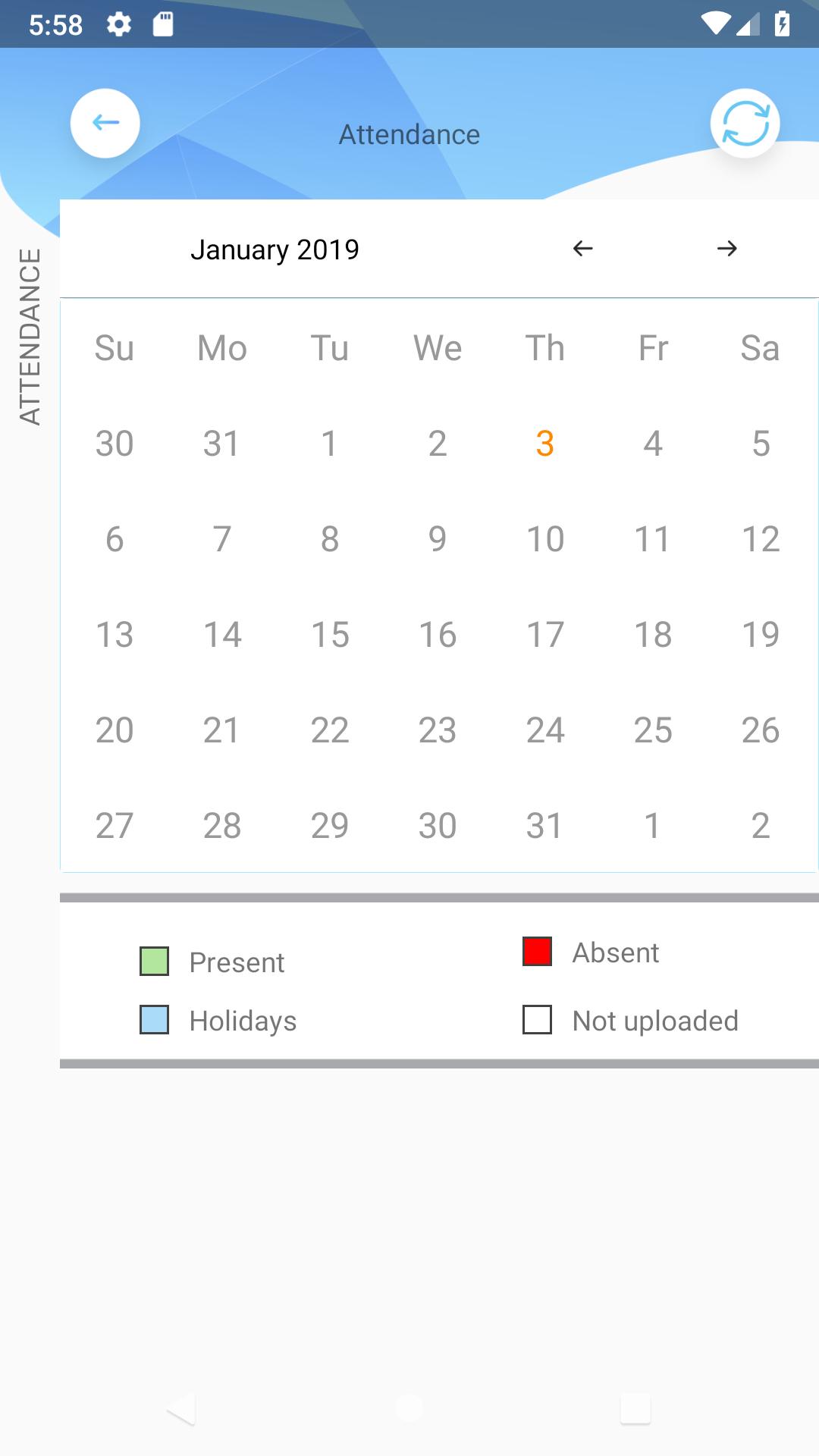The image showcases a calendar interface, presumably from a smartphone, displaying detailed information at 5:58 with a nearly full battery icon shown in white. Dominating the display is the word "Attendance" in the center, accompanied by an upside-down triangle icon to the right. Below this, there are navigation circles: one white circle with a blue left-pointing arrow, and another white circle with looping arrows denoting a refresh option. The calendar is set to January 2019, with left and right arrows for navigating between months.

Beneath the title, the calendar layout includes abbreviated day headers: SU (Sunday), MO (Monday), TU (Tuesday), WE (Wednesday), TH (Thursday), FR (Friday), and SA (Saturday). Under Sunday, the dates listed are the 6th, 13th, 20th, and 27th, while under Monday, the dates are the 31st of the previous month, then the 7th, 14th, 21st, and 28th of January.

At the bottom, there are four color-coded squares indicating different attendance statuses: Green for "Present," Blue for "Holiday," Red for "Absent," and White for "Not Uploaded." This structured and visually organized interface provides a comprehensive overview of attendance tracking for January 2019.